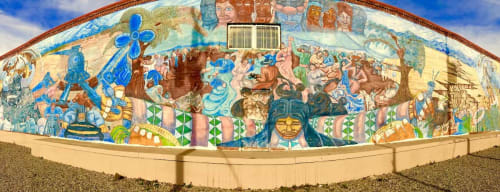The vibrant mural, captured in a close-up fish-eyed lens shot, adorns the side of a building and showcases an intriguing array of characters and details. Dominated by an array of beautiful, multicolored hues—primarily blues, yellows, browns, and greens—the mural's focal point is a serene image of a woman with brown skin, wearing an elaborate headdress and gazing downward. Adjacent to her features a dark-haired man with a goatee, dressed in what appears to be a black robe, his head bowed in a prayerful gesture. Surrounding these central figures are a multitude of other faces and characters, including a row of eight diverse portraits at the top center, each depicting people of different races, colors, and genders. Also interspersed throughout the expansive artwork are large blue flowers, abstract elements, trees, possibly a railroad and car, fan blades, and various animals. The top of the mural is bordered by a distinctive red tile trim and has a vent in the middle, while the bottom features a cream-colored ridge and the foreground includes a gravel area with sprouting weeds. Overhead, the mural is framed by a blue sky filled with wispy, fluffy white clouds, adding a dreamlike quality to the entire scene.